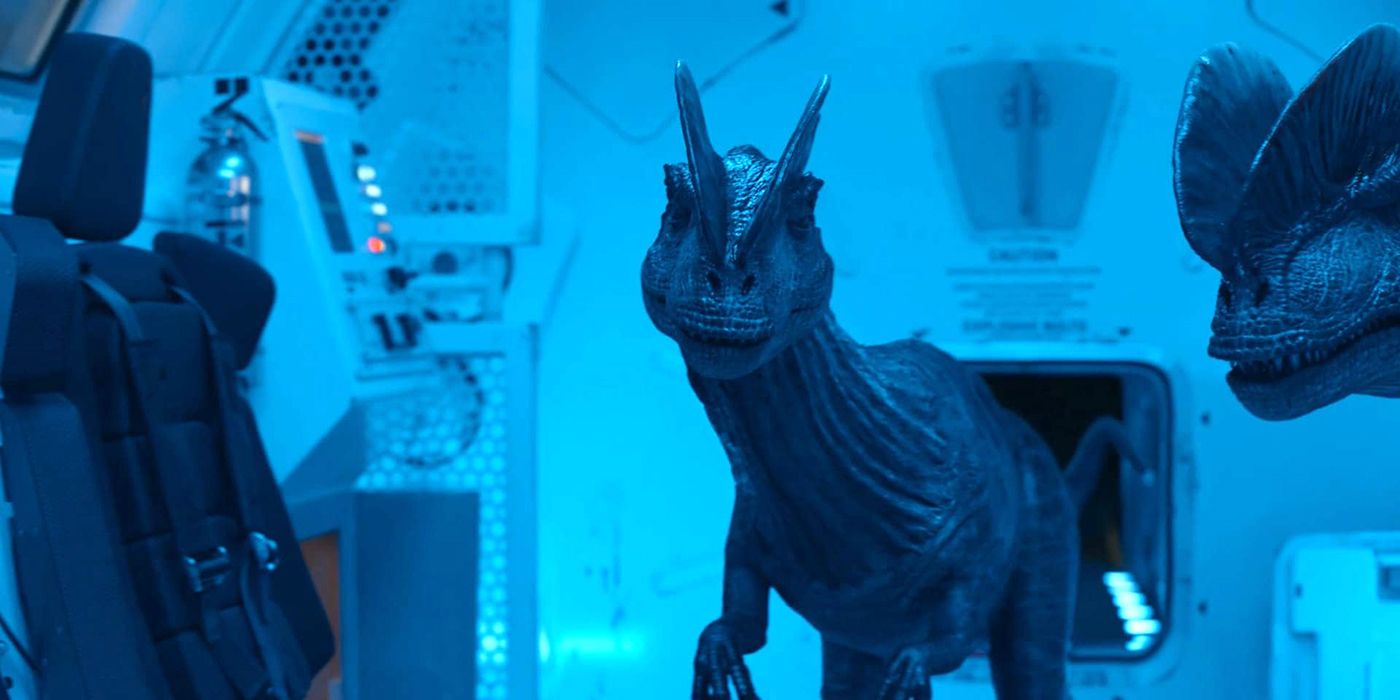The image portrays two dinosaur-like creatures inside what appears to be a spacecraft or aircraft, bathed in a blue filter. The central figure of the image is a dinosaur situated in the middle, facing the camera directly. On the right side, another dinosaur's head is peeking into the frame from the edge. The environment suggests an interior space with metallic elements and aviation components. To the left, there is a seat equipped with buckles and a harness, oriented towards the right. In the background, a metallic cylinder adds to the high-tech, ship-like atmosphere of the scene.